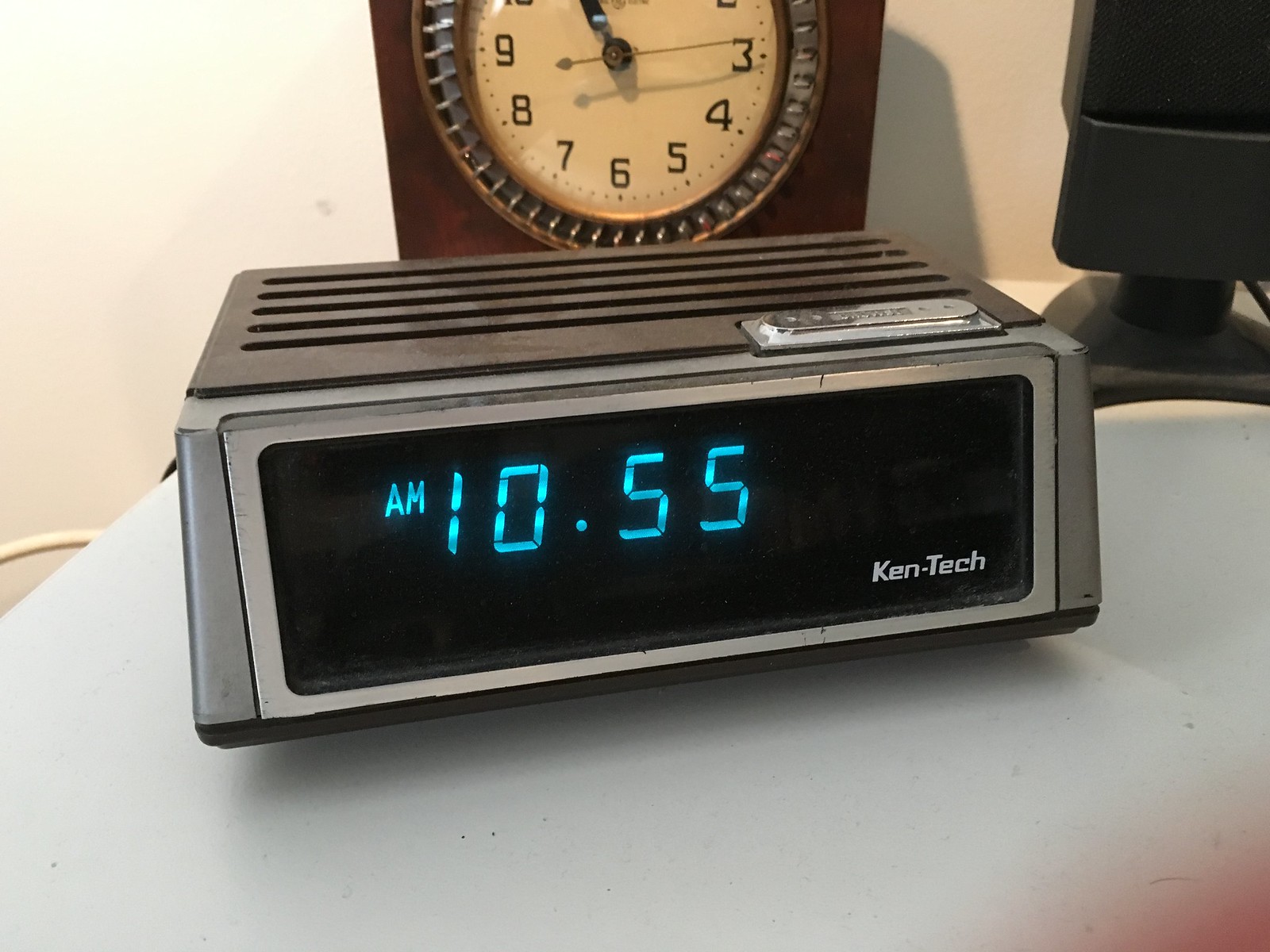The image captures a retro 1980s scene featuring two distinct clocks set against a white veneer surface, probably a nightstand. The focal point is an old-fashioned digital alarm clock with a rectangular box shape. Its top showcases a faux wood grain finish with vent-like grills, while a silver frame surrounds its black screen. The time displayed is 10:55 a.m. in bright blue LED numerals, and the bottom of the screen bears the manufacturer’s name, "Ken-Tech". A white power cable extends from the clock, emphasizing its vintage design. 

In the background, there's a beige wall, a partially visible black speaker or microphone on a stand, and another old clock. This secondary clock features a brown wooden frame, a silver-patterned face, and black Art Deco-style numbers and hands. The overall setting and objects evoke a nostalgic feel, transporting viewers back to a different era.